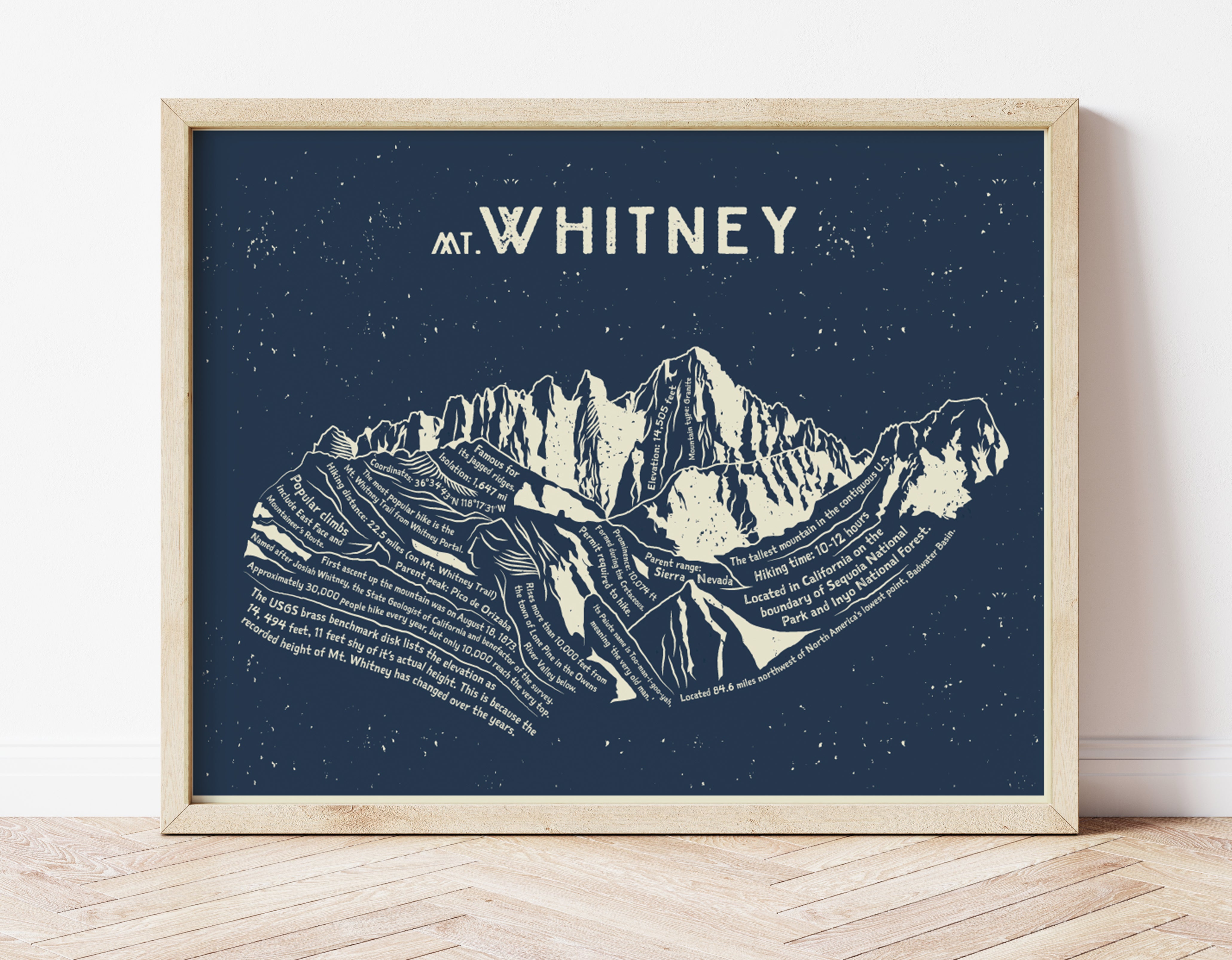The image depicts a decorative framed artwork featuring Mount Whitney. The wooden frame has a light whitish or cream color, beautifully complementing the dark blue background of the illustration. At the top of the artwork, the text "Mount Whitney" is prominently displayed in off-white letters. The central graphic showcases a detailed rendering of the mountainous terrain, accompanied by various informative texts. These annotations describe Mount Whitney as the tallest mountain in the contiguous United States and provide intriguing details such as its coordinates (36°34′43″ N), its location on the boundary of Sequoia National Park and Inyo National Forest, and its parent range, the Sierra Nevada. The illustration further notes that the mountain is famous for its jagged ridges, with the popular Mount Whitney Trail starting at Whitney Portal, which has a hiking time of 10 to 12 hours. The dark blue background features small white dots resembling stars, giving the impression of the mountain floating in a night sky. The artwork is leaning against a white wall, and the floor beneath it has a herringbone wood pattern.